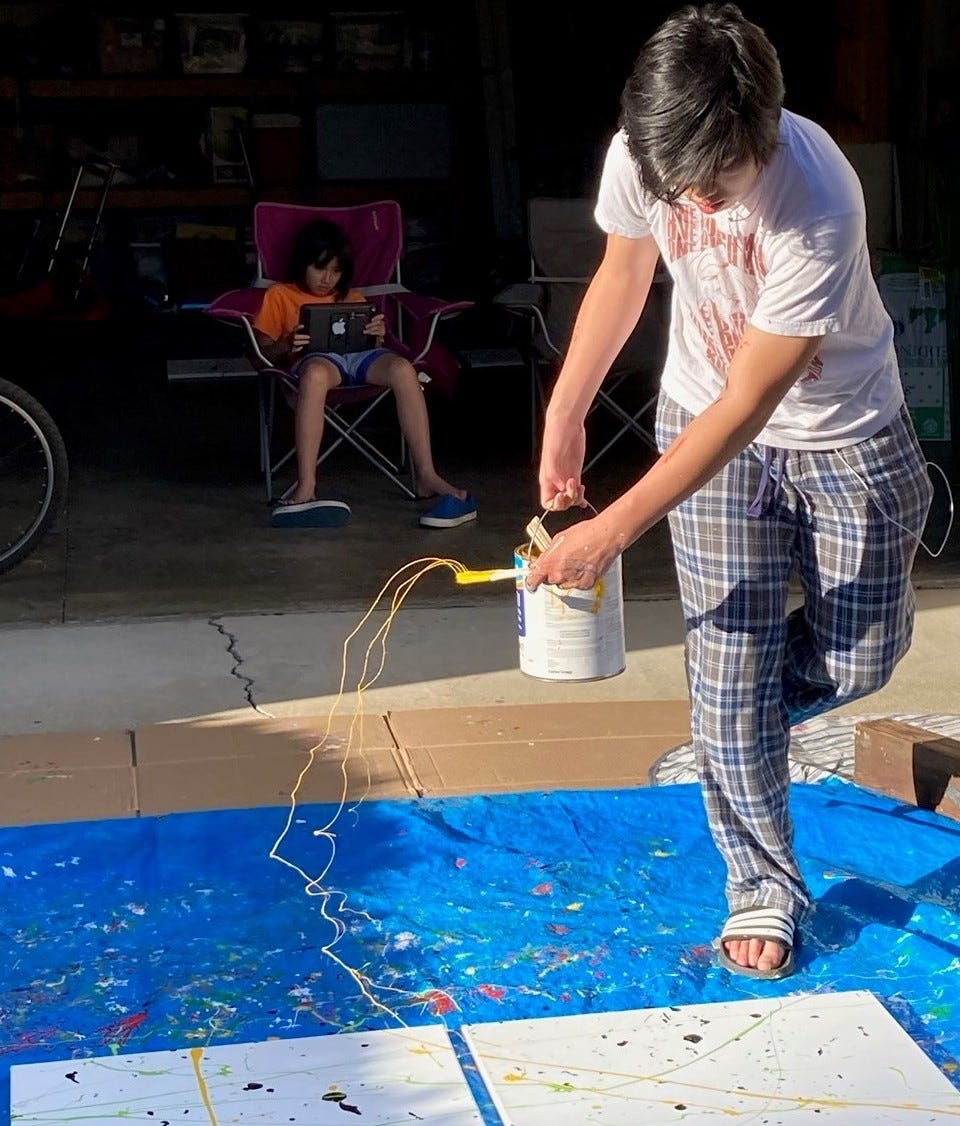In this detailed image, a teenage boy, dressed in plaid blue pajama pants and a white short-sleeve t-shirt with iPhone headphone cords emerging from underneath, is actively engaged in an artistic endeavor. He is positioned over two large white canvases laid out on a protective blue tarp, situated on a cement driveway. The boy holds a bucket of paint in his left hand and a paintbrush drenched in yellow paint in his right hand, slinging the vibrant color onto the canvases, producing a dynamic splatter effect. In the background, inside a garage, a younger boy sits absorbed in his iPad, seated on a red folding chair. The scene is subtly anchored by the presence of a bike tire on the left side of the photo.